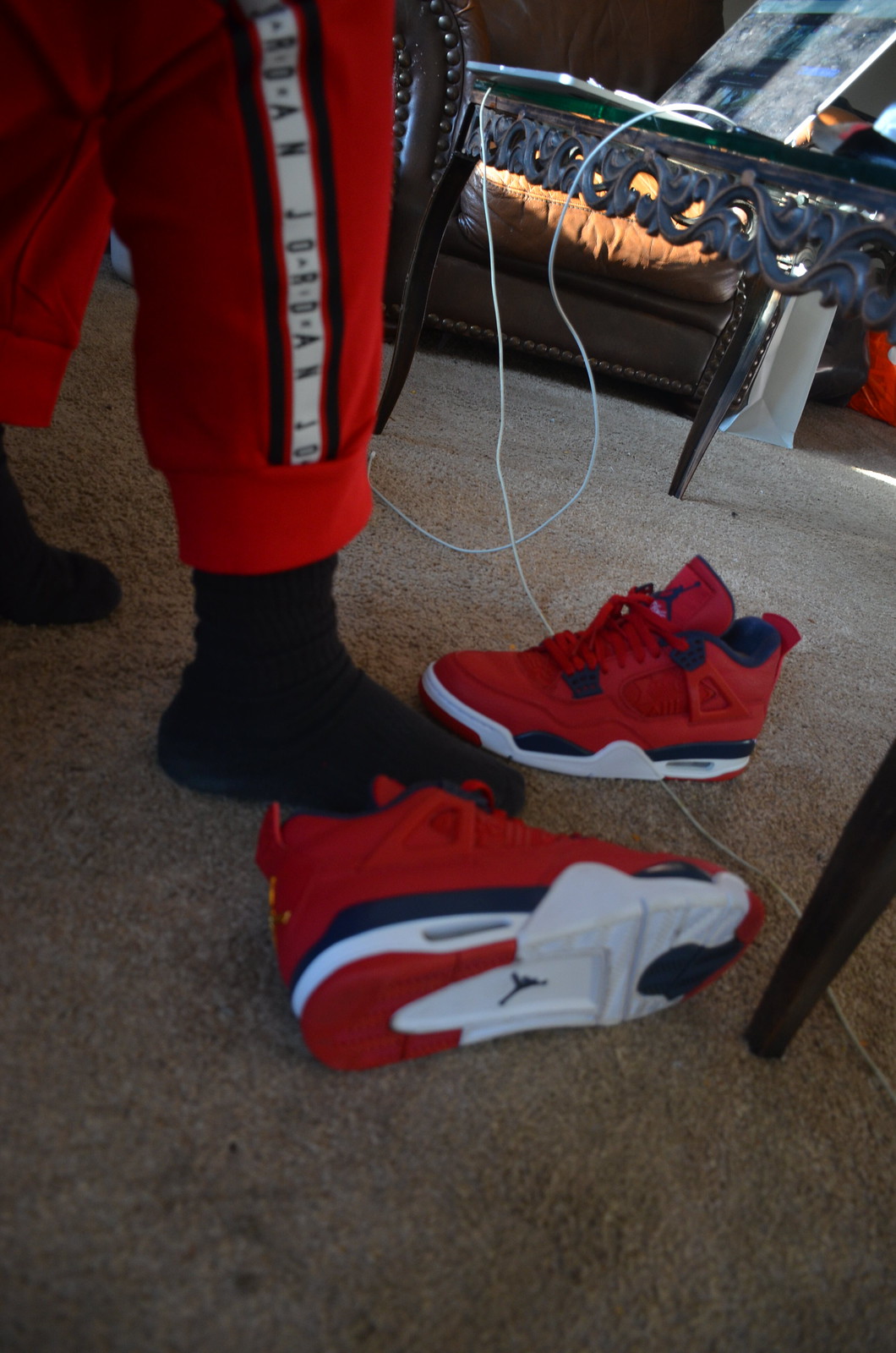In this color photo taken inside a room, we see a person's legs from the knees down standing on a beige carpet. The individual is wearing solid black socks and red Air Jordan sweatpants with a white stripe running down the leg that reads "Jordan" in black. Beneath the person's feet, there are a pair of red, black, and white Air Jordan sneakers. One shoe is tipped over, revealing its white sole with the Jordan logo, while the other shoe rests flat on the somewhat dirty carpet.

In the background, we can see a brown leather armchair adorned with beads, positioned against a white wall. In front of the person, there is a black metal coffee table supporting an open, thin laptop. The laptop has multiple white cords hanging from it, with one trailing to the right and the other to the left, the latter appearing to be a charging cable with a lightning connector not plugged into anything.